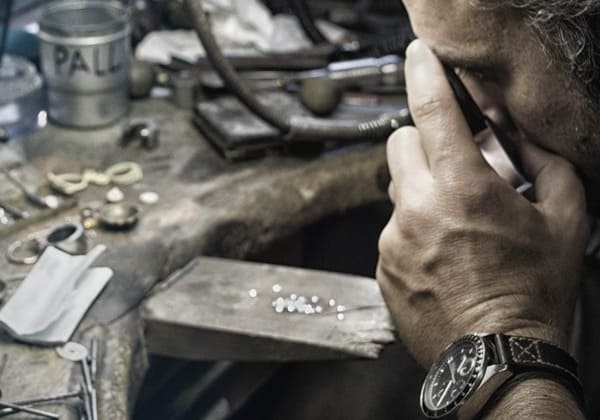The photograph features a Caucasian man in a workshop setting, captured as he peers through a magnifying glass at an array of small, shiny stones—likely diamonds—laid out before him. The man, identifiable by his salt-and-pepper hair, is partially visible with his left hand raised, prominently displaying a wristwatch with a cloth band. He stands next to a countertop with a complex texture, possibly made of stone or wood. This countertop holds various items including paper, metal apparatuses, and a silver pail marked with the text "P-A-L-L." To his right is a narrow shelf attached to the counter, which holds additional small stones, slightly blurred in the background but still discernibly part of his meticulous work environment.